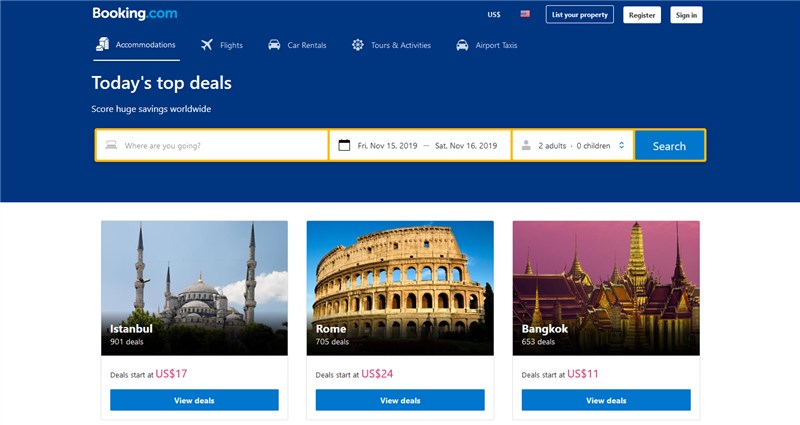This is a screenshot of the Booking.com website homepage. The top of the page features a navigation bar with a US currency icon, a link to list your property, a registration link, and a sign-in link. Below these options is another set of links categorized into Accommodations, Flights, Car Rentals, Tours & Activities, and Airport Taxis.

The page prominently displays a banner that reads "Today's Top Deals" with a subheading, "Score Huge Savings Worldwide." Beneath this banner, there's a comprehensive search box divided into four sections: the first section allows you to input your destination, the second section lets you select your travel dates, the third section is for specifying the number of adults and children traveling, and the fourth section contains the search button to execute your query.

Additionally, this specific page showcases three featured destinations with associated deals, all listed in US currency. The first listing is for Instanbul with deals starting at $17, the second for Rome with deals starting at $24, and the third for Bangkok with deals starting at $11.